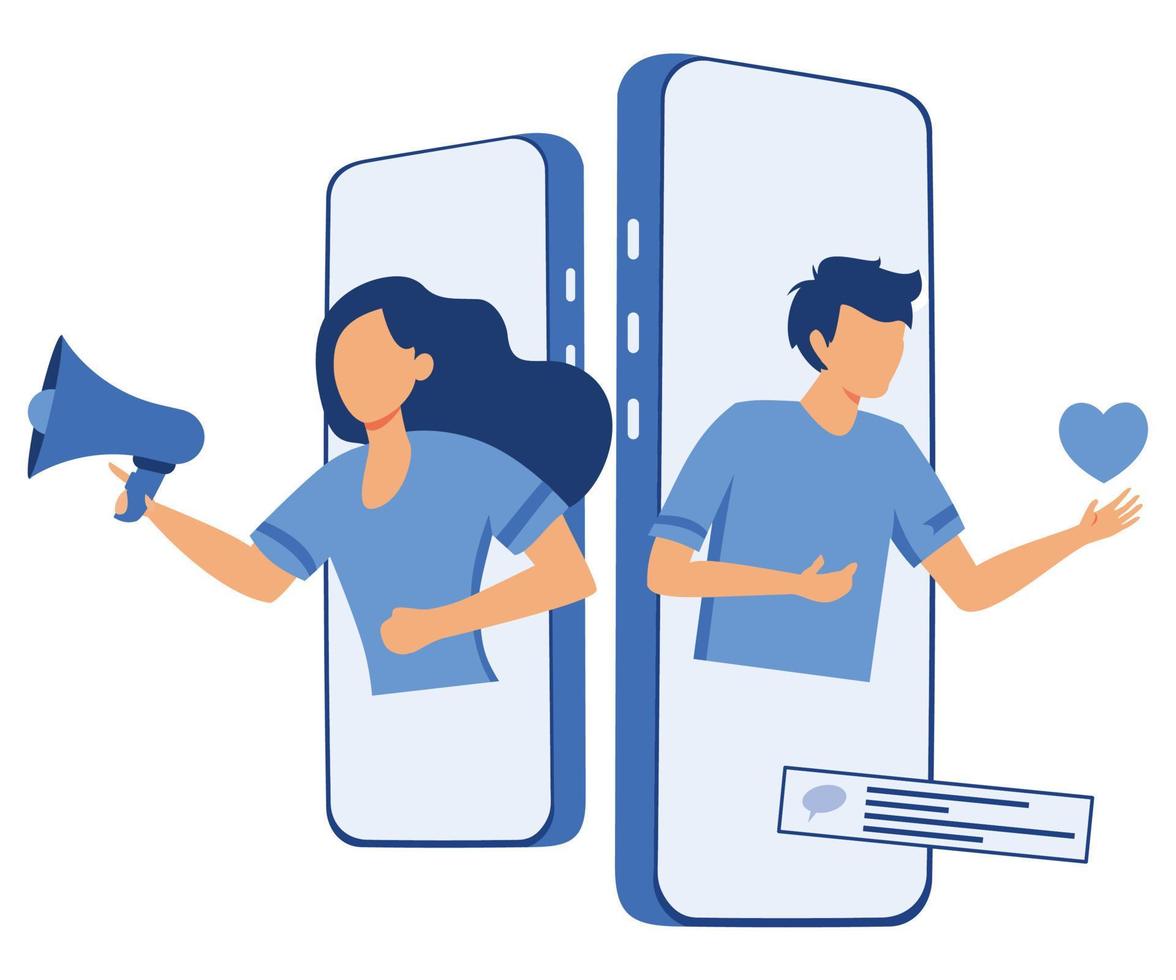This image is a digital illustration resembling an app interface, possibly for social media or a dating profile. On the left, a smaller smartphone displays an abstract cartoon of a woman with flowing, blue hair. She has a peachy-brown complexion and wears a blue shirt while holding a blue megaphone. The illustration is highly stylized, lacking facial features but clearly depicting her head, long hair, and torso.

On the right, a larger smartphone features a similar abstract drawing of a man with short, dark hair. He is clad in a blue shirt and holds a floating blue heart in his left hand while extending his right arm across his body. Below him is an indecipherable text message within a speech bubble, signifying an incoming message. The entire composition uses a blue color palette, tying the characters and elements together, and could be promoting a new smartphone app or feature.